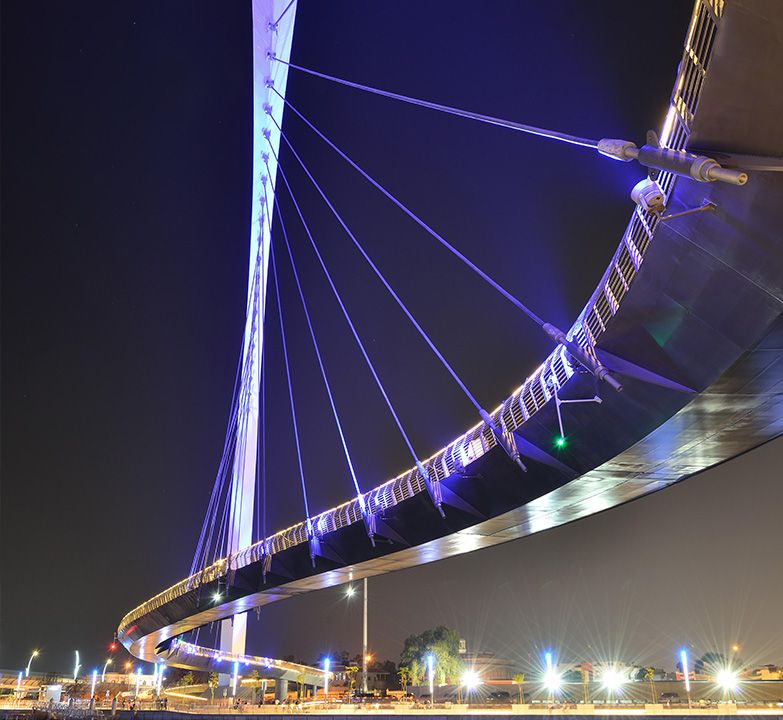The image captures a dramatically lit suspension pedestrian bridge at night, suspended by numerous cables from massive, perforated metal beams and arching structures. The bridge, composed of polished and brushed stainless steel, gracefully curves and snakes its way over a river in a large city. Neon hues bathe the scene in vibrant colors, creating an almost surreal ambiance. Viewed from below, the shot extends from the bottom middle to the top right corner, emphasizing the intricate suspension cables and the sweeping arc of the structure. At the bottom of the image, city lights and street lamps illuminate a bustling, suburban area with two or three people working around the bridge, adding a sense of scale and activity to the scene. The colorful lights of the bridge cast a blue hue over the entire landscape, making the architectural marvel appear even more striking.